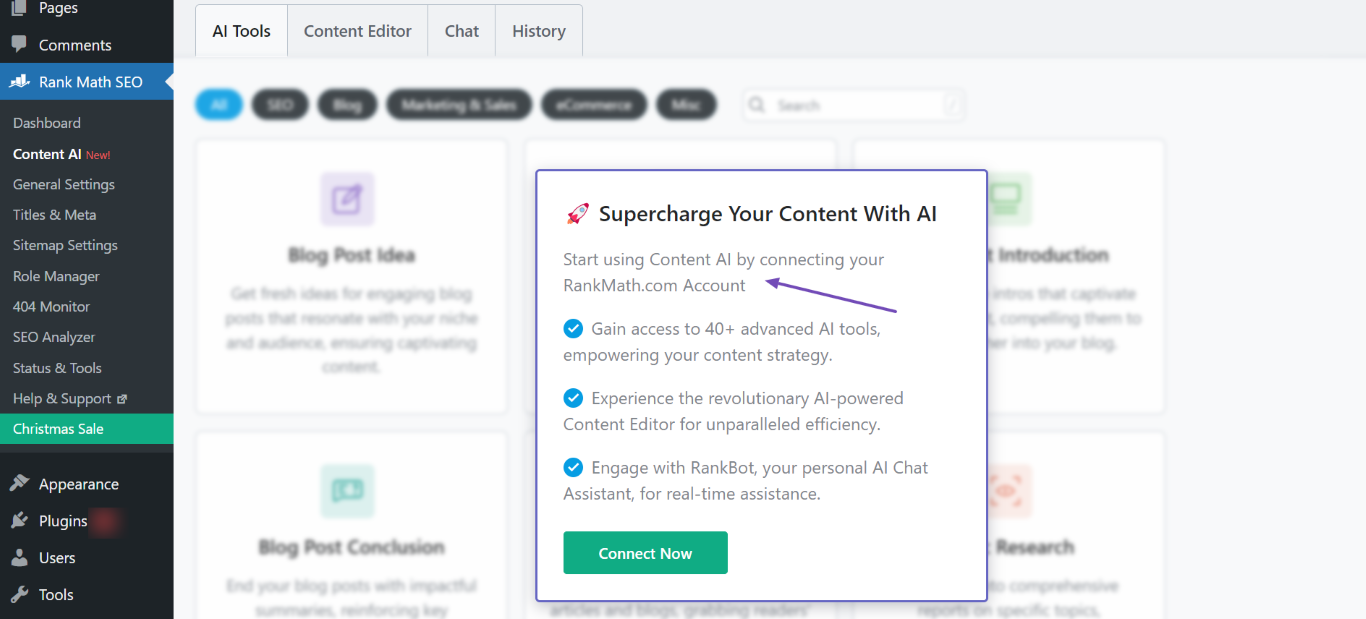The image depicts a webpage interface with a black background featuring a navigational sidebar on the left side. The sidebar menu is presented in a gray font and includes the following options from top to bottom: "Pages," "Comments," "Rank Math SEO," "Dashboard," "Content AI (New)"; the "New" tag is highlighted in red and the text in white. Further down, the menu lists "General Settings," "Titles and Meta," "Sitemap Settings," "Role Manager," "404 Monitor," "SEO Analyzer," "Status and Tools," "Help and Support," "Christmas Sale," "Appearance," "Plugins," "Users," and "Tools."

On the main section of the page, the selected tab is "Rank Math SEO." Across the top, additional tabs are shown: "AI Tools," "Content Editor," "Chat," and "History." A prominent pop-up window overlays the interface, urging users to "Supercharge your content with AI." This pop-up encourages users to "Start using Content AI by connecting your rankmath.com account" and gain access to "40+ advanced AI tools." The features listed in the pop-up include "Empower your content strategy," "Experience the evolution AI-powered content editor for unparalleled efficiency," and "Engage with Rank Bot, your personal AI chat assistant for real-time assistance." Each feature is accompanied by a blue circular bullet point with a white check mark inside it. At the bottom of the pop-up window, a green button labeled "Connect Now" is prominently displayed. Additionally, a purplish-blue arrow points toward the "Start using Content AI by connecting your Rank Math account" prompt, drawing the user's attention to this call to action.